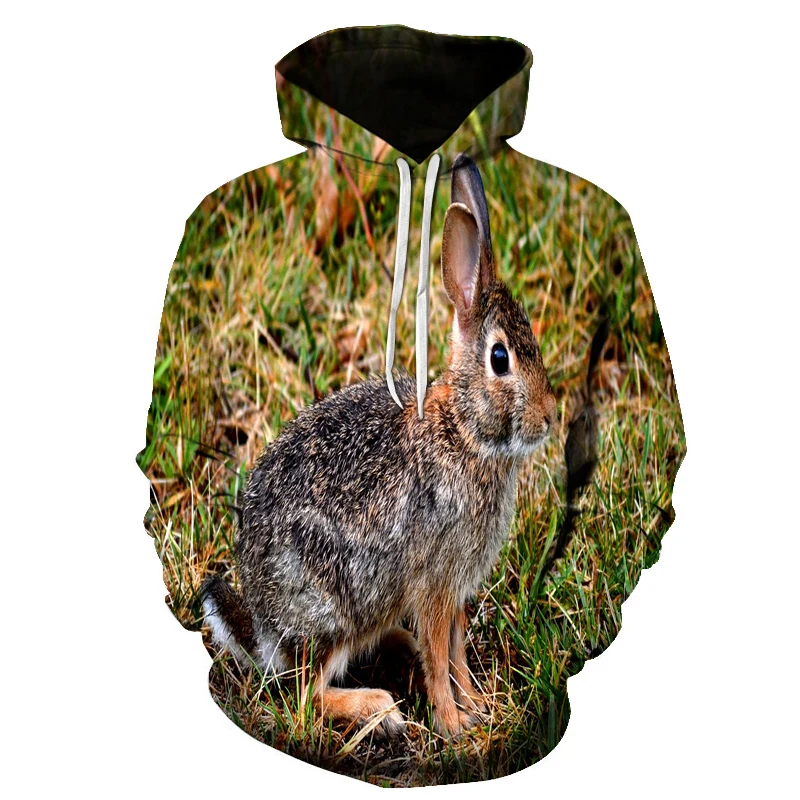This image features a custom-made pullover hoodie adorned with a realistic, albeit slightly warped, depiction of a wild rabbit amidst green and brown grass. The hoodie includes white pull strings hanging from the hood, which is black on the inside. The design covers the entirety of the hoodie, presenting a continuous mural-like scene. The rabbit is prominently displayed from a profile view, showcasing its black eye, light brown nose and legs, white and darker brown fur on its back, upright ears, and a bushy black and white tail. There is no background in the image, only the hoodie with its detailed rabbit and grass design. The quality of the print appears low, detracting somewhat from the overall effect.